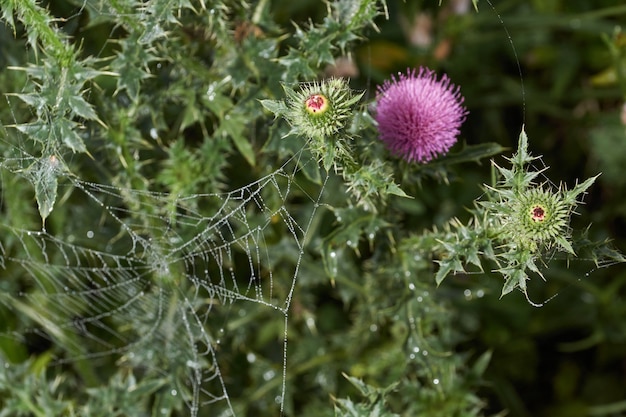This photograph captures a vibrant plant with a delicate spiderweb stretched across its sharp, needle-like leaves. The prominent feature is a striking pinkish-purple flower, resembling a spiky ball, providing a strong contrast against the lush green foliage. Surrounding this primary bloom, there are smaller green buds that also have spiky exteriors, with hints of yellow and red towards their centers, suggesting they may not yet have fully bloomed. The leaves of the plant are pointed and resemble cacti or spiky weeds, enhancing the plant’s rugged appearance. The spiderweb, possibly glistening with morning dew, is intricately woven among the tiny branches and adds a touch of ethereal beauty to the scene. The background becomes blurred with additional greenery, bathed in soft sunlight, emphasizing the plant's captivating details in the foreground.